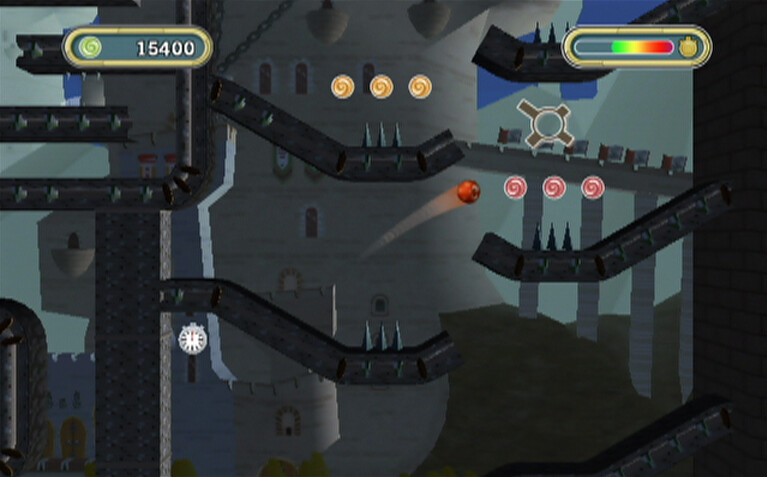In this still image from a video game, a sprawling gray castle dominates the background. The castle features numerous skinny windows with arched tops, some of which lead to small, balcony-like spaces. Intricate details such as a series of winding, maze-like pipes are prominently displayed. These pipes have sharp bends and are menacingly adorned with metal spikes, contributing to the foreboding atmosphere. At the top of the screen, there are interface elements including a section that displays the player's score and another that indicates the health status.